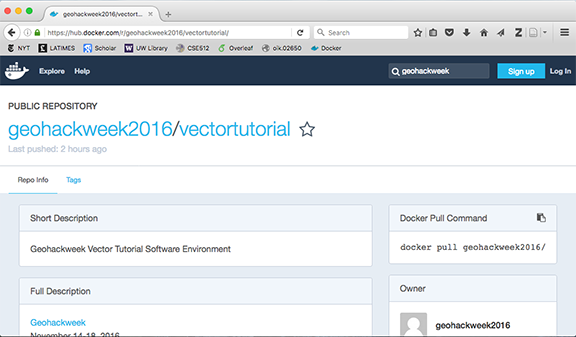A screenshot of a web browser displays the URL "https://hub.docker.com/r/geohackweeks/k2016vectortutorial" in its address bar. The browser interface includes a prominent blue bar at the top. Below this bar, a repository page for Geohackweeks 2016 Vector Tutorial is shown. The page features a search bar with the text "Explore, Help, Geohackweeks" and two blue rectangular buttons labeled "Sign Up" and "Login."

The repository information indicates that it is a public repository titled "geohackweek 2016 / vector tutorial" and includes a hollow star icon. It notes that the repository was last pushed two hours ago. The interface also has a navigation line with options including "Repo Info," "Tags," "Short Description," and "Full Description," all related to the Geohackweek software environment.

On the right side of the page, there are instructions for pulling the Docker image, including the command "docker pull geohackweek 2016/vector tutorial." The owner of the repository is specified as "geohackweek 2016" in a grayed-out square. The overall layout suggests it is a detailed webpage viewed within a browser.